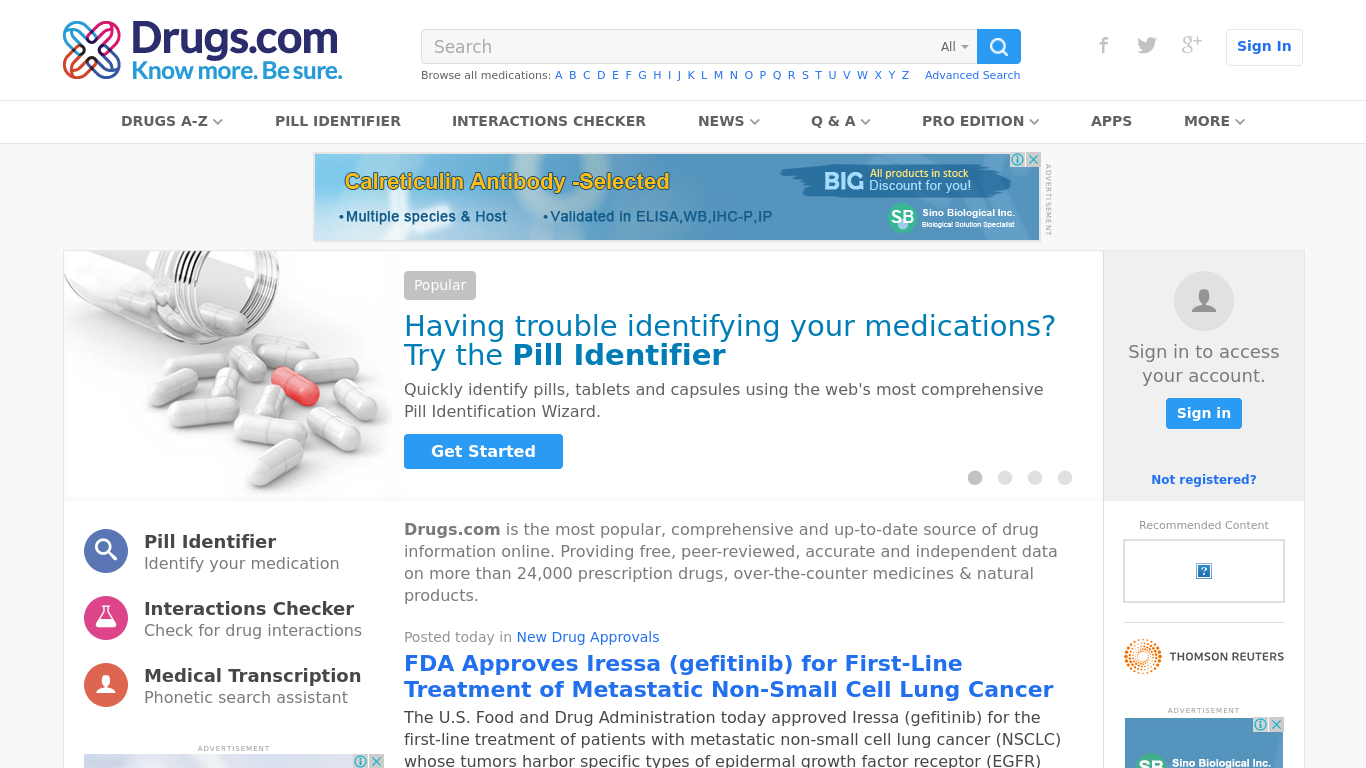This image is a detailed screenshot from the Drugs.com website interface, featuring various elements and options for user navigation. The focal point of the page is a graphic overlay of two intersecting pills colored blue, burgundy, and light blue, accompanied by the text, "Be Sure." A prominent search bar with an all-blue button is situated to the right, next to social media icons for Facebook, Twitter, Google+, and a sign-in option.

Above the main menu, users are invited to "Browse All Medicines," providing an A to Z index for advanced search capabilities. The main navigation menu includes tabs labeled: Drugs A-Z, Pill Identifier, Interactions Checker, News, Q&A, Pro Edition, Apps, and More.

A prominent advertisement for "Calrexulin, Antibody Selected, Multiple Species and Host Validated by ELISA WB-IHC-PIP" is displayed below the menu. Next, a 3D rendering depicts a bottle of pills, with white pills scattered on a table and a single red pill in the center.

Further down, the page offers tools like the "Pill Identifier" to help users identify their medication, and an "Interactions" checker for drug interactions. It features a small icon of a person's face to symbolize user consultations, and various small icons populate the left margin. To the right, highlighted sections such as "Popular" and "Having Trouble Identifying Your Medications?" prompt users to try the Pill Identifier tool with a "Get Started" button.

Below this, text emphasizes the popularity of the site and includes a section headed "New Drug Approvals" in blue text. For example, the FDA-approved "Iressa (gefitinib) for the first-line treatment of metastatic non-small-cell lung cancer" is mentioned. Sign-in options and a couple of small advertisements are also present on the right side of the page, facilitating user engagement and navigation.